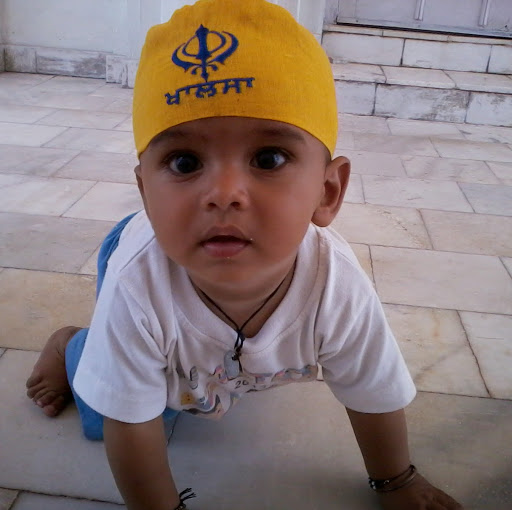In a pristine, minimalist white room featuring a white marble floor extending towards the viewer, white walls, and a couple of marble steps leading to a white wooden door, a baby crawls on all fours, directly facing the camera. The background includes white and gray marbled tiles that add subtle texture to the scene. The infant, appearing to be male, captivates with his big eyes and black pupils. He dons a bright yellow cap adorned with a deep blue logo of three swords and text written in an unfamiliar language. The baby is dressed in a white t-shirt with black lettering and wears a distinct black necklace adorned with a small silver dog tag. His wrists are accessorized with black armbands, and a glimpse of his blue pants peeks out from behind him. The baby's right foot is partially visible as he looks inquisitively towards the camera, creating a compelling and detailed portrait amidst the serene setting.